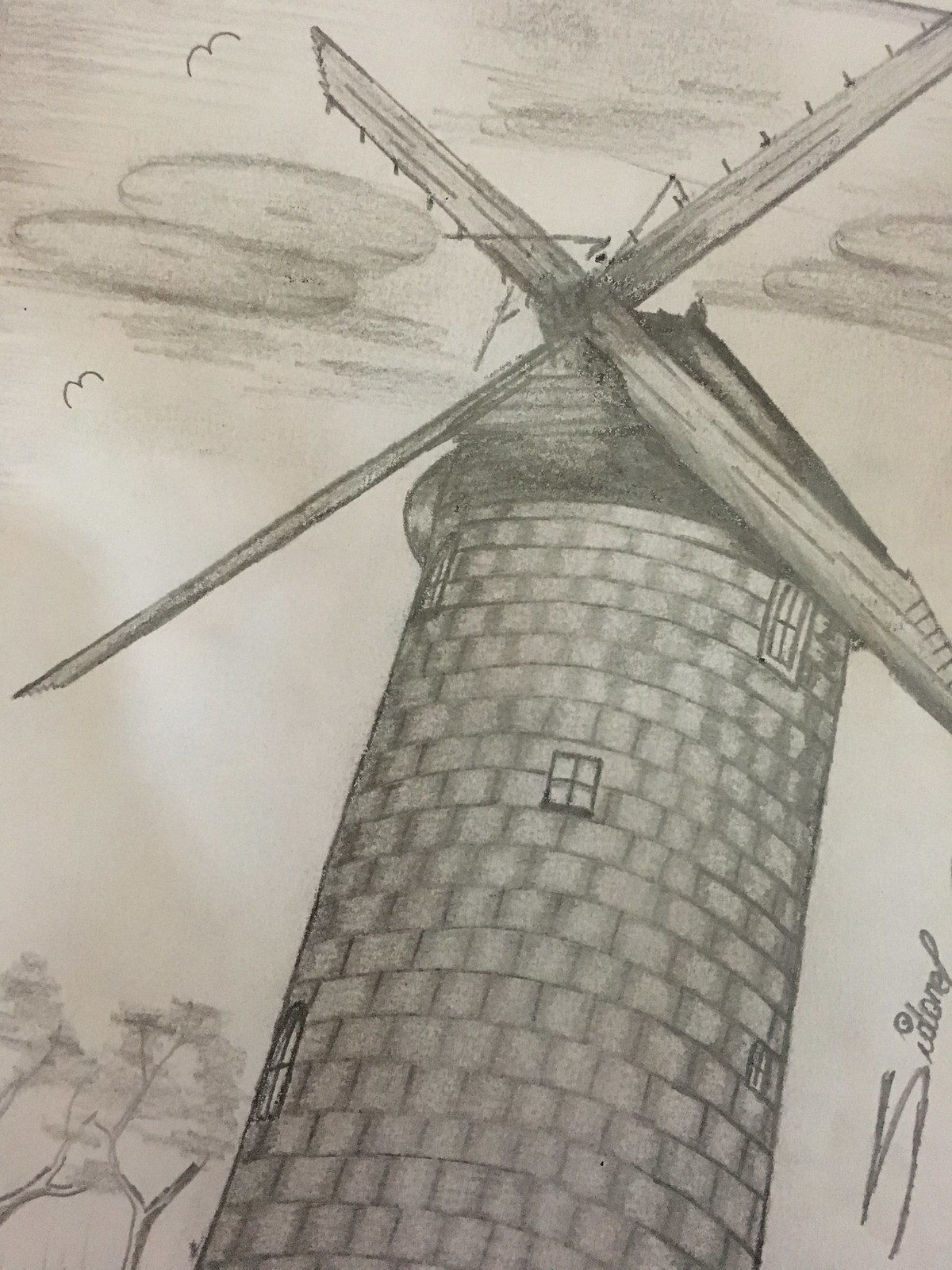The image is a detailed pencil drawing of a tall windmill constructed from small, square brick pieces. The drawing, rendered in shades of black and white, is viewed from a bottom-up perspective. The windmill features several small windows, each about a fourth of an inch tall, distributed along its height. At the top, the tower has a rounded edge, from which long, slender blades extend, forming a distinctive X shape characteristic of windmills. In the background, shaded clouds fill the sky, and small squiggly lines represent birds in flight. On the bottom left, there are trees with visible branches, adding to the scenic composition. The artist’s signature, possibly reading "Siderell," is clearly marked in the bottom right corner, further authenticating the work.